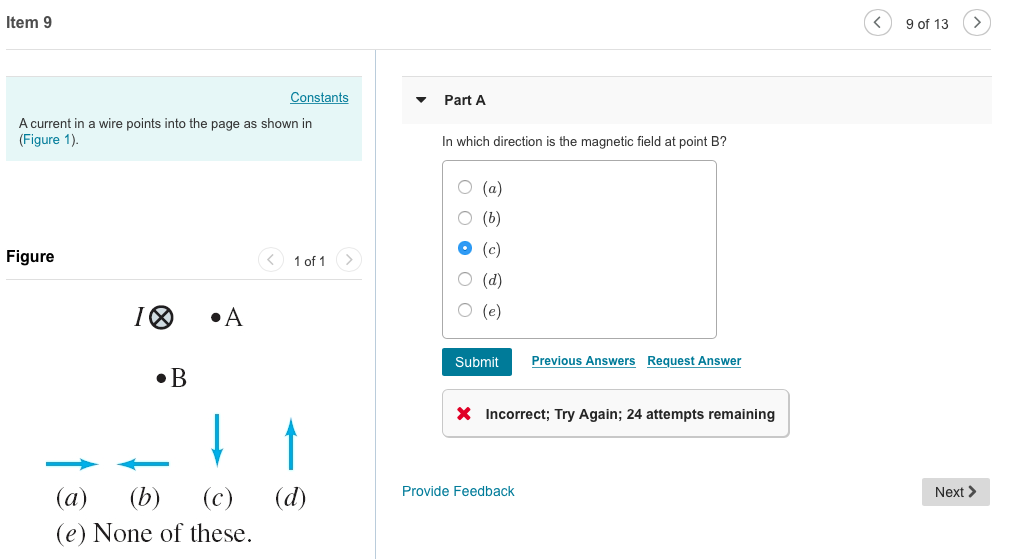A detailed caption for the described image:

---

The image displays a segment of a digital assessment, currently at item 9 out of 13, as indicated in the top right corner. Navigation arrows for moving to the previous or next question are also present. The visible part of the question appears to contain a diagram labeled as Figure 1, showing a wire with a current flowing into the page, represented by the standard X symbol. The diagram includes two points labeled A and B, along with several blue arrows pointing left, right, up, and down, which are labeled as answer choices A, B, C, D, and an option E for none of these.

The question prompt reads: "In which direction is the magnetic field at point B?" The respondent has to choose from one of the blue arrows designated by the letters A, B, C, D, or E. In this instance, the respondent selected option C, which corresponds to the downward-pointing arrow. After submitting their answer, the system feedback indicated that the response was incorrect and prompted the user to try again, noting that they have 24 attempts remaining. The unusual allowance of 24 attempts despite there being only five answer choices is also noted.